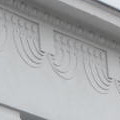This is a very small, postage-stamp-sized daylight photo capturing a highly detailed and ornate Romanesque architectural feature on the white side of a building. The image shows a portion of a wall beneath an eave or overhang that extends outward. This overhang contains intricate sculpting in the molding, featuring alternating circles and lines that appear like balls. Below the molding, the design cascades into swirling semi-circles that resemble curtains being pulled back and tied off. These patterns create a dynamic, wave-like effect with lines that emphasize the parting curtain motif. Additionally, the sculpted design includes rectangles and arches that nearly touch but remain distinctly separate, highlighting the craftsmanship. Although primarily white, a slight angle of the roof on the top right side introduces a subtle, light blue hue, possibly due to lighting. This highly decorative section of the building's exterior showcases a patterned, repetitive arrangement of these elaborate elements.